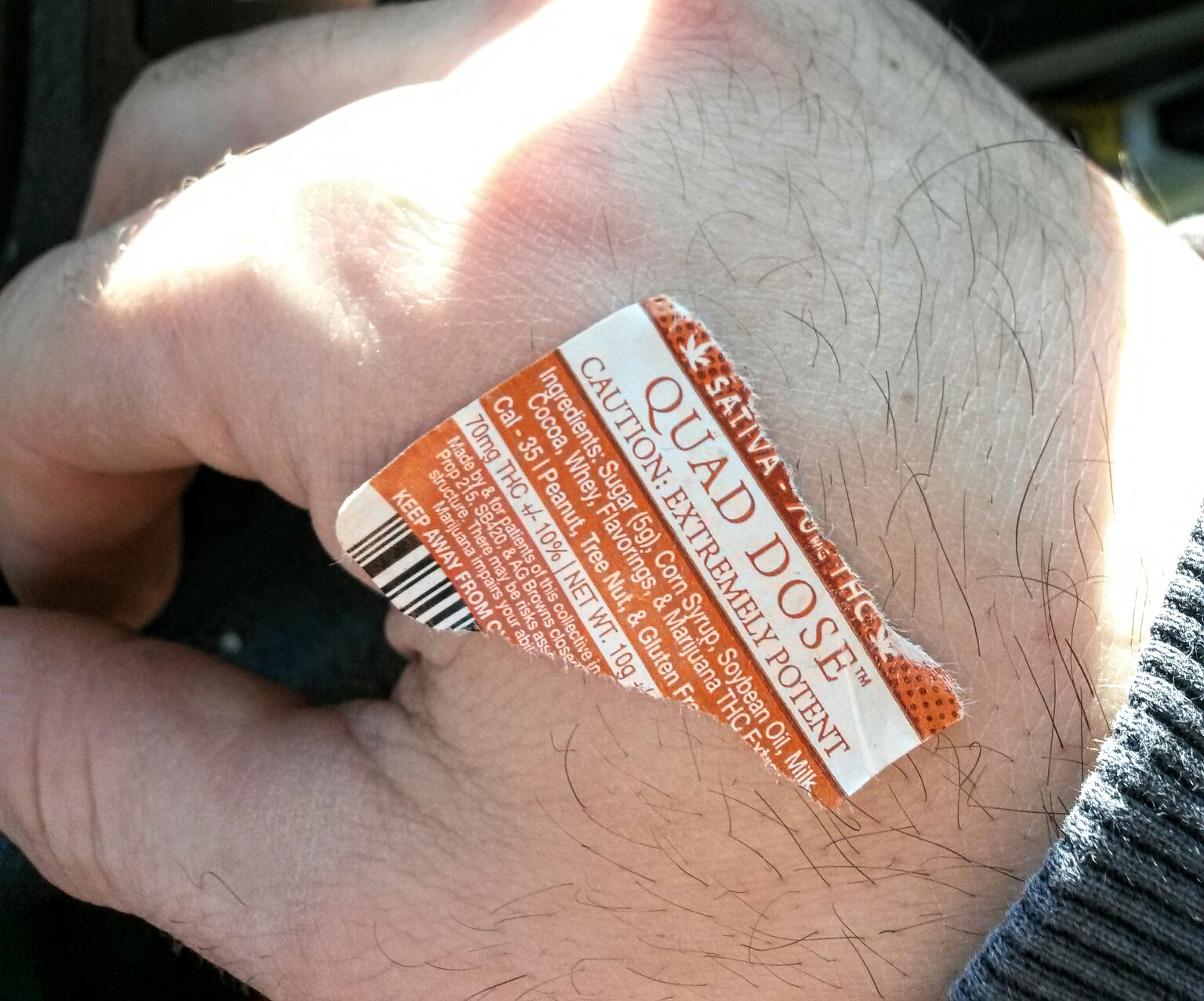This is a close-up image of a white man's hairy hand, positioned in front of what appears to be a car dashboard, suggesting he's sitting inside a vehicle. The man's grey sweater sleeve is partially visible. A partially torn product sticker is adhered to the top of his hand, between the thumb and pointer finger. The sticker details a potent cannabis-infused product with the label reading "Quad Dose™ Sativa 70 mg THC," and includes a caution about its potency. The list of ingredients are: sugar (5 grams), corn syrup, soybean oil, milk, cocoa, whey, flavorings, and marijuana (THC extract). It also mentions being calorie-conscious with 35 calories and notes being free from peanuts, tree nuts, and gluten. The sticker specifies the product is "made by and for patients of this collective." Although parts of the text are torn and missing, it suggests keeping the product away from children.